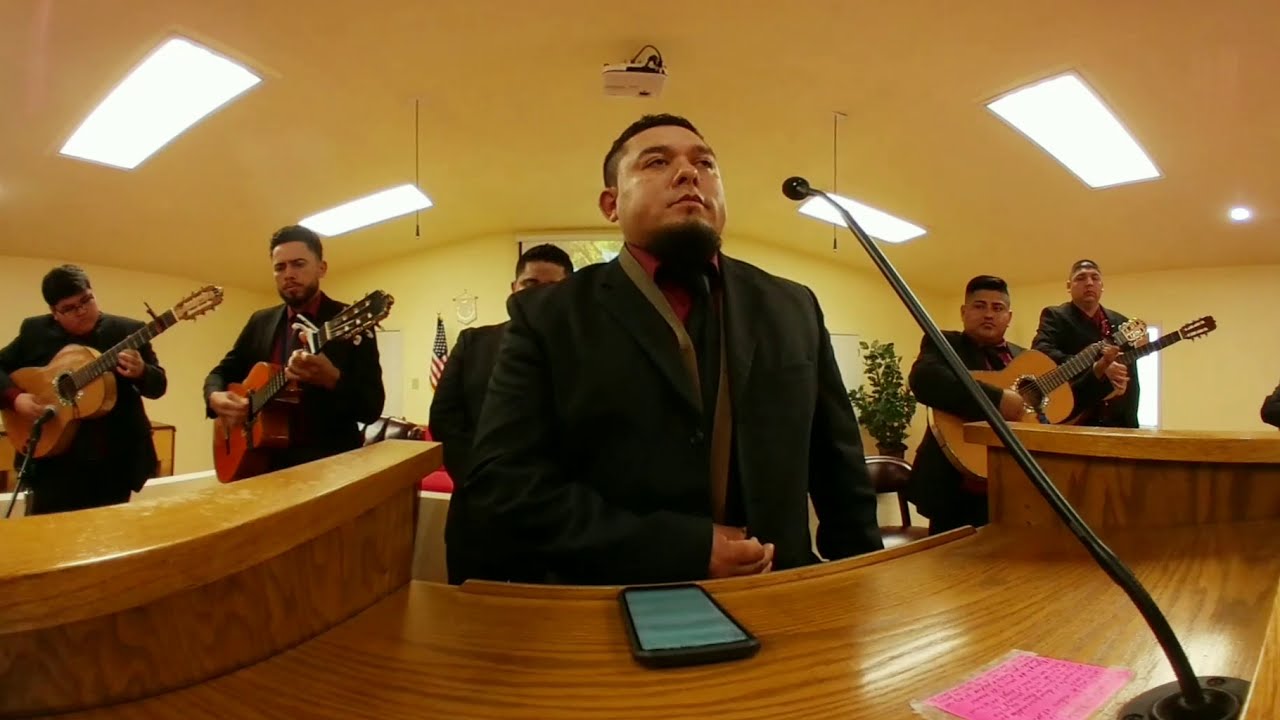This interior color photograph captures a six-member band, potentially of Mexican or Spanish heritage, dressed in coordinated outfits of black suit jackets, red collared shirts, and black ties. The central figure, a man with short dark hair and a goatee, stands at a podium made of bright orangish-brown wood, adorned with a smartphone and a pink post-it note beneath a tall black microphone stand. The podium curves outward in the middle and has wooden sides extending to the left and right. He stands confidently with one arm across his chest and the other by his side. Behind him, arranged in a room with yellow walls and overhead rectangular light panels, are five other men, each holding and playing large wooden acoustic guitars with black fittings. They mirror the central figure's attire. In the room, additional details include an overhead white projector, an American flag on a pole at the back left, and a ficus tree with green leaves. The setting's precise nature is nuanced, possibly within a church or a community hall, enhancing the formal yet intimate ambiance.